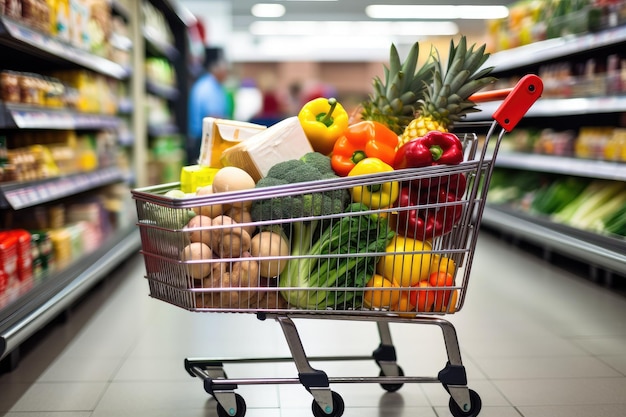The photograph depicts a grocery store aisle with a cream-colored tile floor. In the center foreground, there is a small silver shopping cart, sized for a child, with a vibrant red plastic handle. The cart is filled to the brim with various fruits and vegetables, including large pineapples, a sizable head of broccoli, and an assortment of bell peppers in yellow, orange, and red. Also visible among the produce are round fruits and vegetables such as tomatoes, potatoes, onions, and possibly oranges. The aisle stretches out into the distance, flanked by fully stocked shelves displaying products in a range of colors—green, yellow, red, and more—adding to the visual richness of the scene. The background is blurred, giving the main focus to the cart, yet one can discern at least one person with black hair and wearing a blue shirt, standing slightly to the left. The overall look of the image, with its muted and slightly blurred background, provides an almost uncanny, computer-generated or rendered feel.